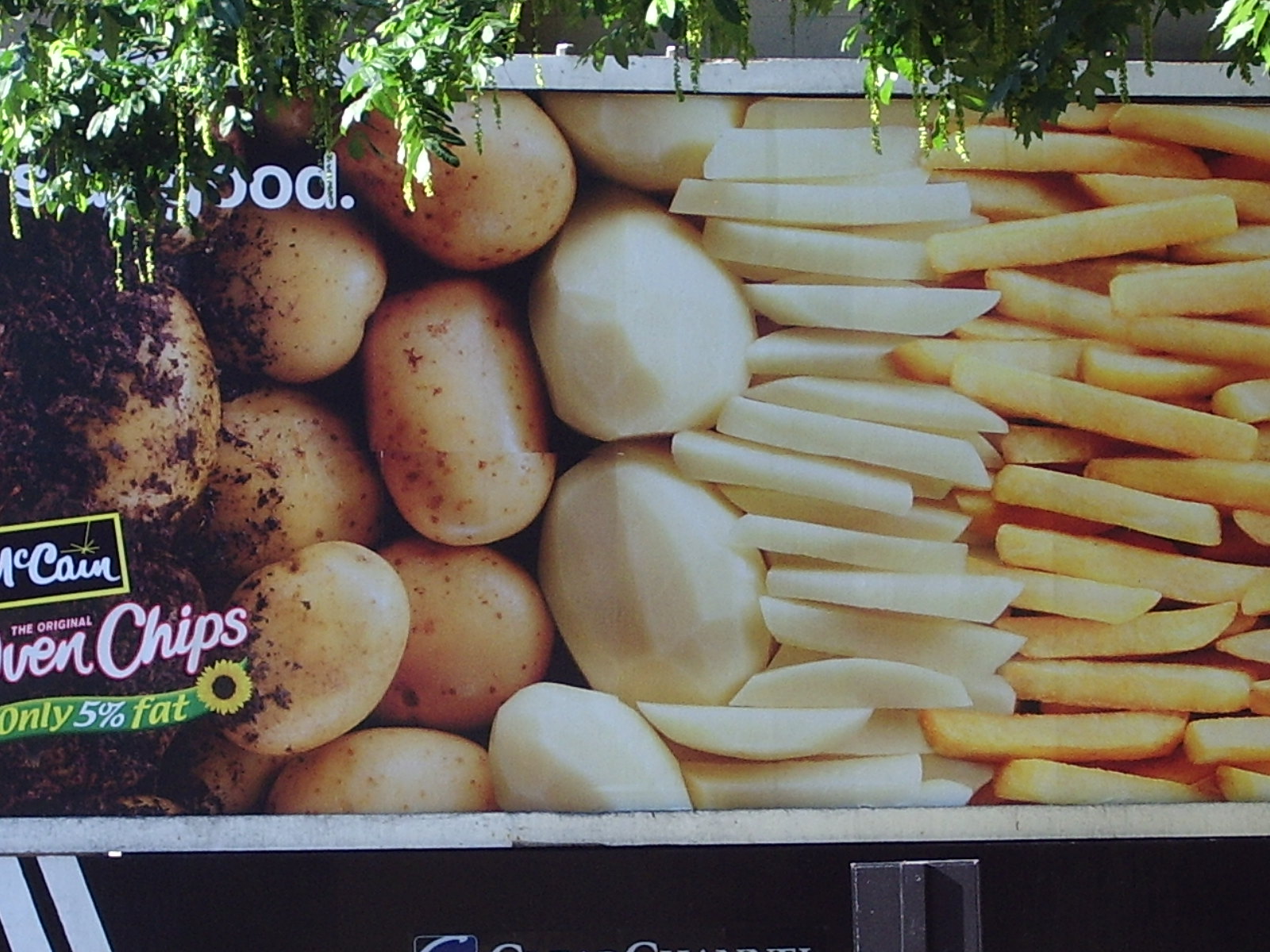The image features a visually organized display of various stages of potatoes and their transformation into French fries. In the bottom left corner, a sign prominently reads, "McCain Chips only 5% fat," partially obscured by some tree branches hanging down. From left to right, the image starts with a patch of dirt filled with whole, unpeeled raw potatoes. Next, there is a section showing a collection of peeled potatoes, followed by another section with these peeled potatoes cut into raw French fries. The progression continues with a row of cooked French fries. The top left corner of the sign has partially hidden text that seems to state "So Good" or a similar phrase, though the view is obstructed by the hanging tree branches. The bottom of the image is marked by a solid black line that runs horizontally from left to right.